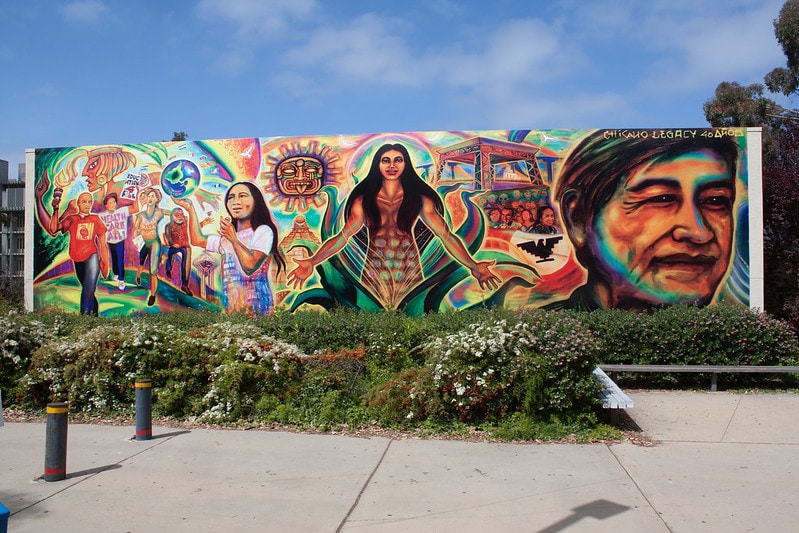The photograph captures an intricately detailed mural displayed on a prominent billboard that spans most of the image from left to right. The mural, vibrant and colorful, sends a powerful message with its richly illustrated elements. On the left side, a group of people are depicted marching together, holding a torch and signs. Behind them, an Egyptian-looking hieroglyphic figure emerges. To the right of this scene, a little girl is seen holding up a marble or sphere. Higher up, an ancient Mayan or Aztec sun crowns a pyramid. Dominating the center, a person with long black hair stands with arms spread wide, with a crowd of people visible under a structure to their right. On the far right, a close-up of a man's face is prominently displayed. Above in the mural, the words "Chicano Legacy" are inscribed, emphasizing its cultural significance.

The mural is set against a bright blue sky filled with fluffy white clouds, enriching the overall scene. In the background, trees with lush green leaves frame the top right corner. The foreground is meticulously landscaped with a variety of white and pink flowers, alongside squared bushes. To the right side of this green area runs a small metal bench, low to the ground, complementing the scene. On the left side, two gray metal pillars with yellow stripes on top and red stripes on the bottom stand on the sidewalk, providing a structural element to the composition. The overall atmosphere is one of intention and care, both in the mural's creation and the landscaping that frames it.